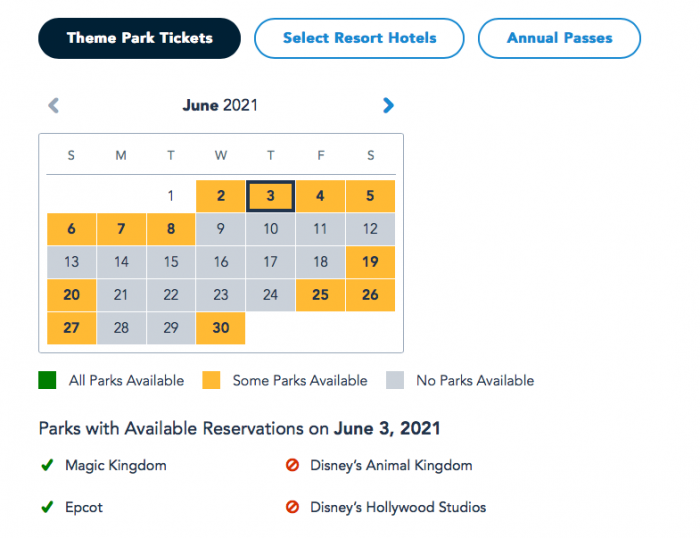The image depicts a Disney reservation calendar for June 2021. At the top of the interface, there are three buttons. The leftmost button is a darker blue and labeled "Theme Park Tickets" in white text. The middle button reads "Select Resort Hotels," and the rightmost button says "Annual Passes."

Below these buttons is a calendar header displaying "June 2021," flanked by a gray left arrow and a blue right arrow for navigation. The calendar itself displays the days of the week abbreviated as "SMTWTFS" along the top row, followed by a grid of the month's days starting with June 1st on a Tuesday and ending with June 30th on a Wednesday.

Dates from June 2nd to June 8th are highlighted in yellow boxes, as well as some additional scattered dates below. Most of the middle dates are shaded gray. A legend underneath the calendar explains the color-coding: a green box indicates "All Parks Available," a yellow box means "Some Parks Available," and a gray box signifies "No Parks Available."

A summary below the legend lists the availability of reservations for June 3rd, 2021. It shows that Magic Kingdom and Epcot are fully available with green checkmarks, while Disney's Animal Kingdom and Disney's Hollywood Studios are unavailable, marked by red crossed-out symbols.